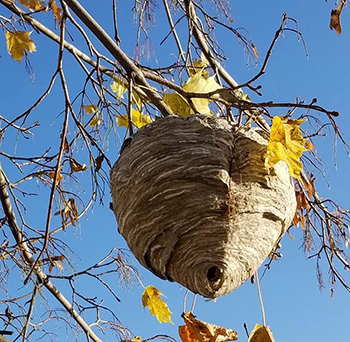This square-shaped color photograph captures an autumn scene, prominently featuring a large paper wasp nest hanging from the end of a branch in a mostly barren tree. The image is taken from a perspective slightly below and to the right of the nest, looking up into an absolutely clear, bright blue sky with no clouds visible. The tree appears to be a maple, as evidenced by a few remaining yellow and brown leaves and some characteristic maple whirligig seeds scattered among the branches. The nest itself, approximately the size of a football, shows distinct shadowing on the left side, making it appear darker, while the right side is more illuminated. At the bottom of the nest, a noticeable hole can be seen. Despite the barren state of the tree and the crisp clarity of the day, there are no insects visible around the nest. The branches surrounding the hive are a mix of white and brown, with some appearing dead, underscoring the late autumn season.